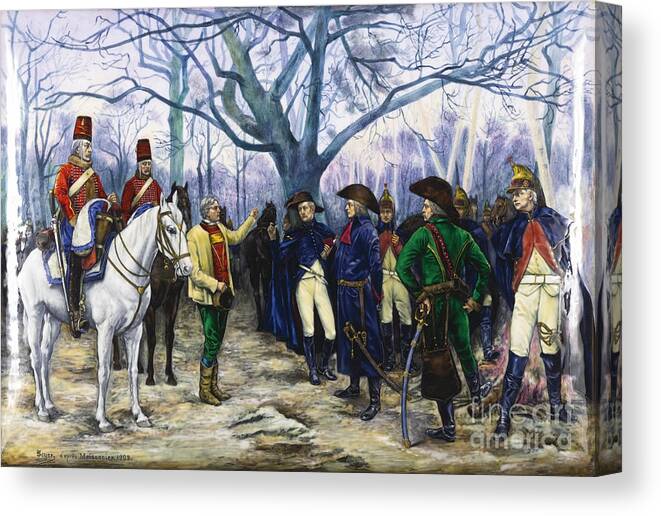The image appears to be a product photo of a high-quality print or painting, available for purchase on a website, with the watermark "Fine Art America" visible in the bottom corner. It depicts a historic scene possibly from the Civil War era or older, characterized by intricate details and a striking composition.

In the background, a sprawling, leafless tree extends its branches over a predominantly white and bluish-gray setting. The foreground features a dirt ground and a group of seven soldiers congregating on the right side. These soldiers are predominantly attired in long blue coats, with one member distinguished by a bright green coat. They wear hats or helmets, some adorned with gold parts, and three of them wear brown hats. Many are equipped with swords, either in hand or attached to their waists.

On the left side, a man dressed in green pants, brown boots, a red shirt, and a yellowish jacket is prominently featured, engaging with the soldiers. He is bareheaded and sports a gold necklace, with his left arm raised as if in the midst of a discussion.

Behind this man, two figures on horseback add depth to the scene. One rides a white horse while the other rides a brown horse. Both riders are clad in distinctive red uniforms with matching fezes that have gold accents, cream sashes, and numerous gold buttons. The entire composition suggests a moment of significant interaction or negotiation between the groups depicted.